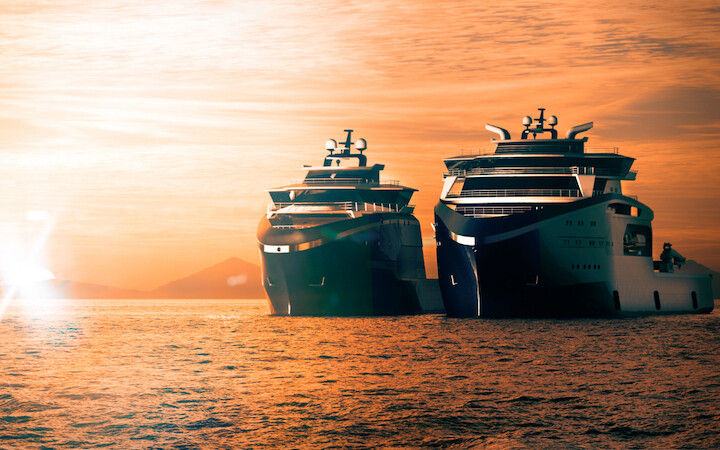The image features two ultra-modern ships, possibly commercial or private yachts, sailing side-by-side in calm waters during a sunset. The ships have sleek, contemporary designs with smooth lines and modern railings. The larger ship is predominantly black with chrome accents, while the smaller one appears to be green. Both vessels are outfitted with advanced features, including stylish components for ventilation. The sun is setting on the left side of the image, casting an orange and red tint over the ocean and sky, contributing to a warm glow that highlights the ships' gleaming surfaces. In the distant background, dark hills or a mountain range add depth to the serene seascape.